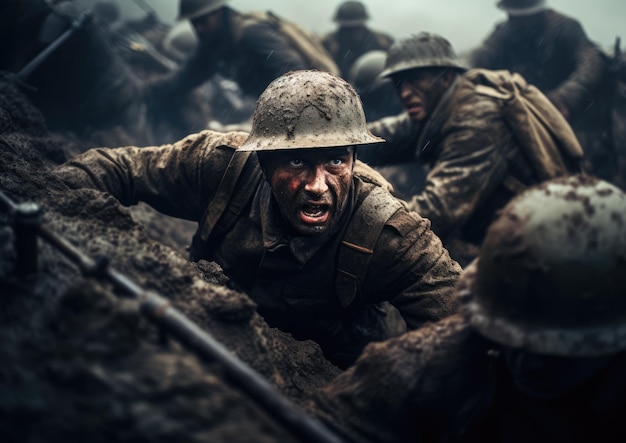The image appears to depict a dramatic scene, likely from a World War I or World War II movie, featuring gritty trench warfare. At the center of the photo, a soldier with a dirt-covered face, wearing a green combat uniform and a hard helmet, is seen lying in a trench amidst the muddy and rain-soaked earth. His focus is directed slightly to the right, suggesting vigilance or anticipation. Surrounding him in the background, numerous other soldiers, similarly clad in military fatigues and helmets, seem poised to emerge from the trench. There is a noticeable helmet lying on the dirt to the right of the central soldier, along with what seems to be a rifle. The chaotic atmosphere is further emphasized by raindrops streaking across the image and the palpable tension among the soldiers, who appear to be receiving orders from a commanding figure. The detailed representation of the muddy conditions, the soldiers’ readiness, and the intense expressions convey the harrowing and gritty reality of battle, indicative of a powerful war film.